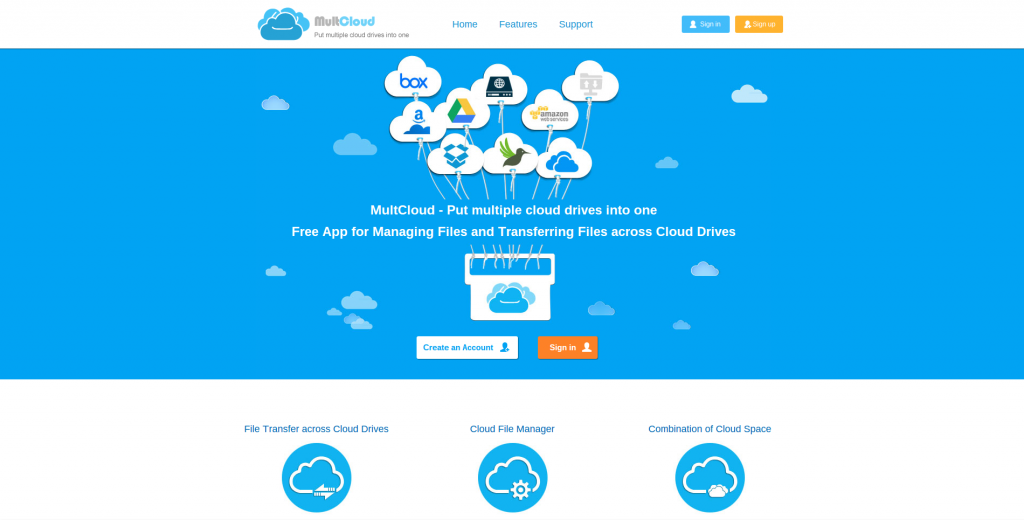This is a cropped screenshot of a webpage with a blue background. The header at the top left of the page is white and features the title "Mole Cloud" with small grey text beneath it. To the left side of the header, there is blue clipart of clouds. Centered in the banner at the top are hyperlinked words in blue: "Home," "Futures," and "Support." On the right side of the header are two buttons: a blue one and an orange one, both with very tiny white text.

The main body of the webpage showcases nine white cloud-shaped balloons with strings attached, resembling cloud-shaped logos mid-hover. These balloons display various company logos, including Box, a recycling symbol, and Twitter, amongst others that are too small to identify clearly. They are centralized on the page, with their strings leading into a box illustrated at the bottom of this section.

Below the cloud balloons, a description reads: "Multi Cloud: Put multiple cloud drives into one free app for managing files and transferring files across cloud drives." Directly beneath, there are two buttons for user actions: a white button labeled "Create an Account" and an orange button labeled "Sign In."

At the very bottom of the page, three cloud icons are displayed. The left icon depicts a white cloud with a lightning bolt, the center icon shows a white cloud with a sun, and the right icon features a white cloud with snow. Each icon includes small blue text above it, though the text is not legible.